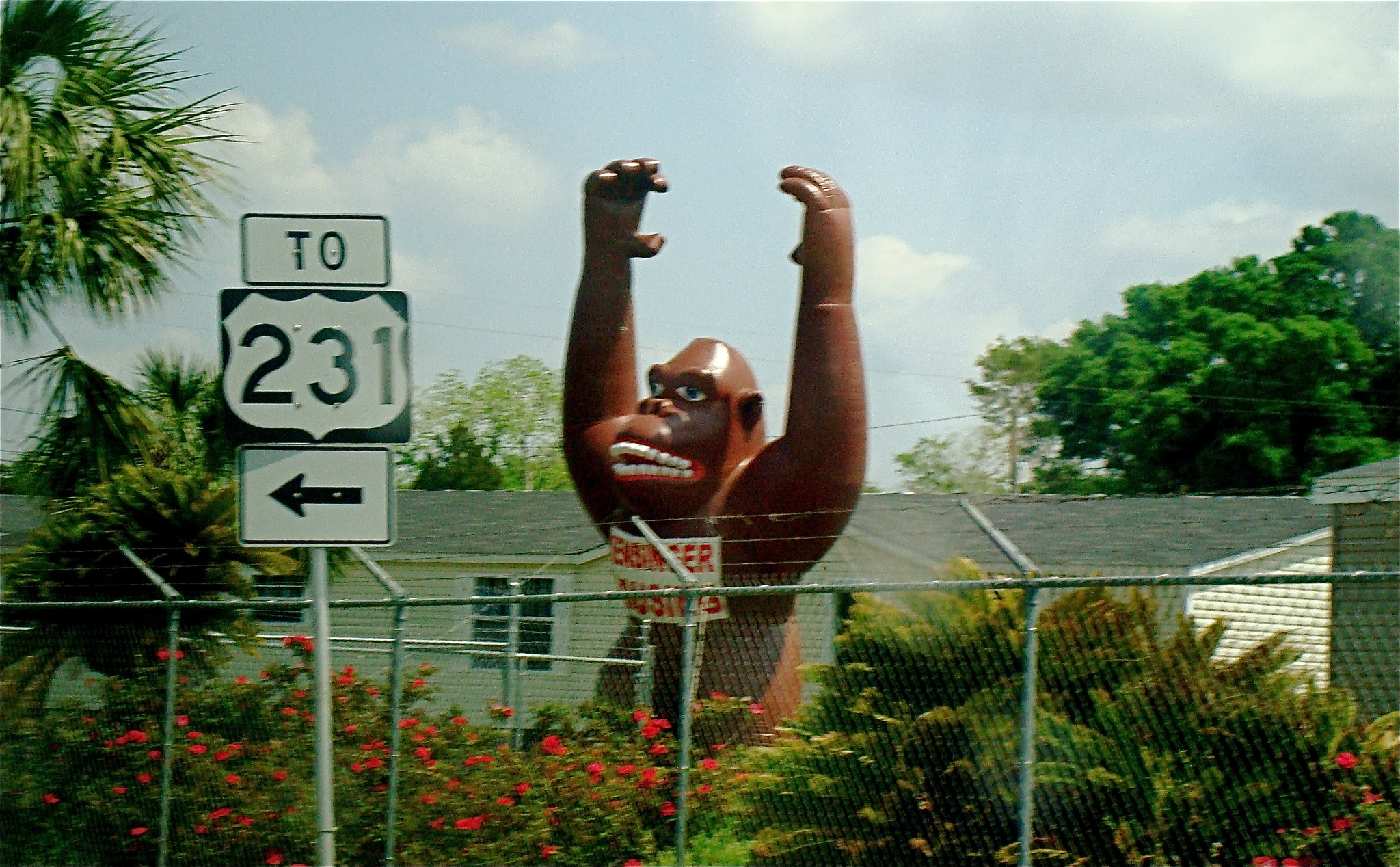In this vibrant outdoor photograph, taken in landscape orientation, the foreground features a chain-link fence adorned with blooming watermelon-colored roses. Directly in front of the fence stands a steel post bearing a red sign indicating Route 231 ahead, with a black arrow emphasizing the direction. Beyond the fence, a colossal plastic gorilla statue dominates the scene, its arms raised menacingly over its head and a scowl etched onto its face, baring its teeth. A white poster with bold red lettering is affixed to the gorilla's chest, partially legible with the words "Busters" and an indistinguishable word ending in "ER." The background showcases a cluster of white buildings with distinct rooftops, interspersed with tall, swaying palm trees and other lush greenery. The blue sky overhead is dotted with fluffy white clouds, adding a cheerful contrast to the surreal scene below.